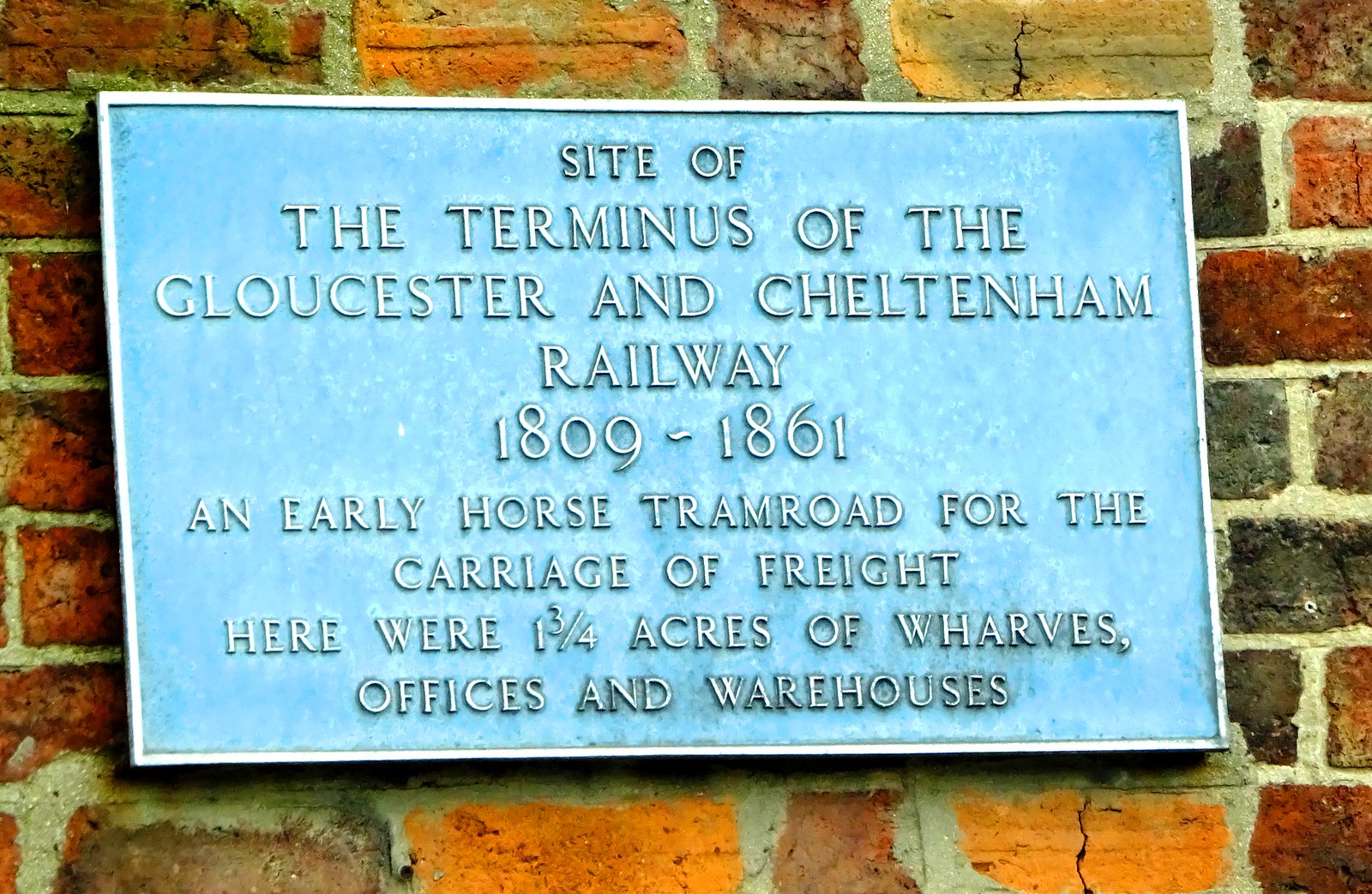The image depicts a close-up of a historical plaque mounted on an exterior brick wall. The brick wall, composed of red, dark gray, orange, and tan bricks separated by light gray mortar, forms a vibrant, textured backdrop. The rectangular plaque, slightly tilted towards the top left corner of the image, has a solid gray border with a weathered, blackened center. The inscription on the plaque reads, "Site of the Terminus of the Gloucester and Cheltenham Railway, 1809 to 1861. An early horse tram road for the carriage of freight. Here were one and three-quarter acres of wharves, offices, and warehouses." This dedication plaque marks the historical significance of the location as a former transportation terminal associated with early freight carriage by horse tram.